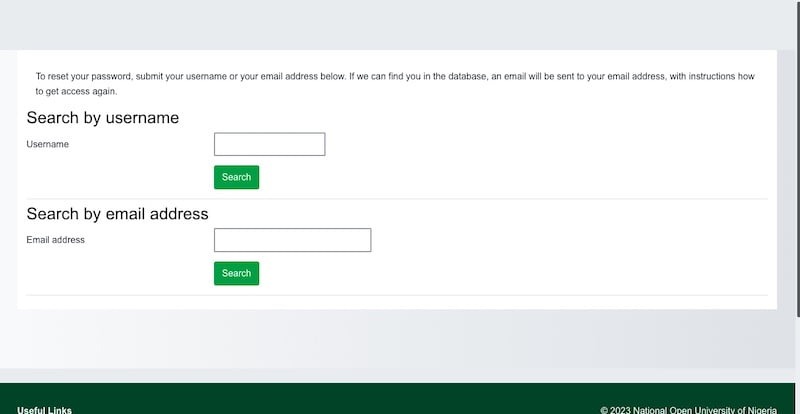This image is a detailed screenshot of a "Forgot Username" webpage from a website. The top of the page provides instructions: "To reset your password, submit your username or your email address below. If we can find you in the database, an email will be sent to your email with instructions on how to get access again."

In the middle section, the page offers two methods to recover your username or password. The first method allows users to search by their username. Here, there is a text box to input the username along with a green rectangular search button labeled "Search" in white font. The second method offers the option to search by email address. Similar to the username section, this method includes a text box to input the email address and an identical green rectangular search button labeled "Search" in white font.

At the bottom right corner of the page, the text "2023 National Open University of Nigeria" is clearly visible, indicating the affiliation of the webpage.